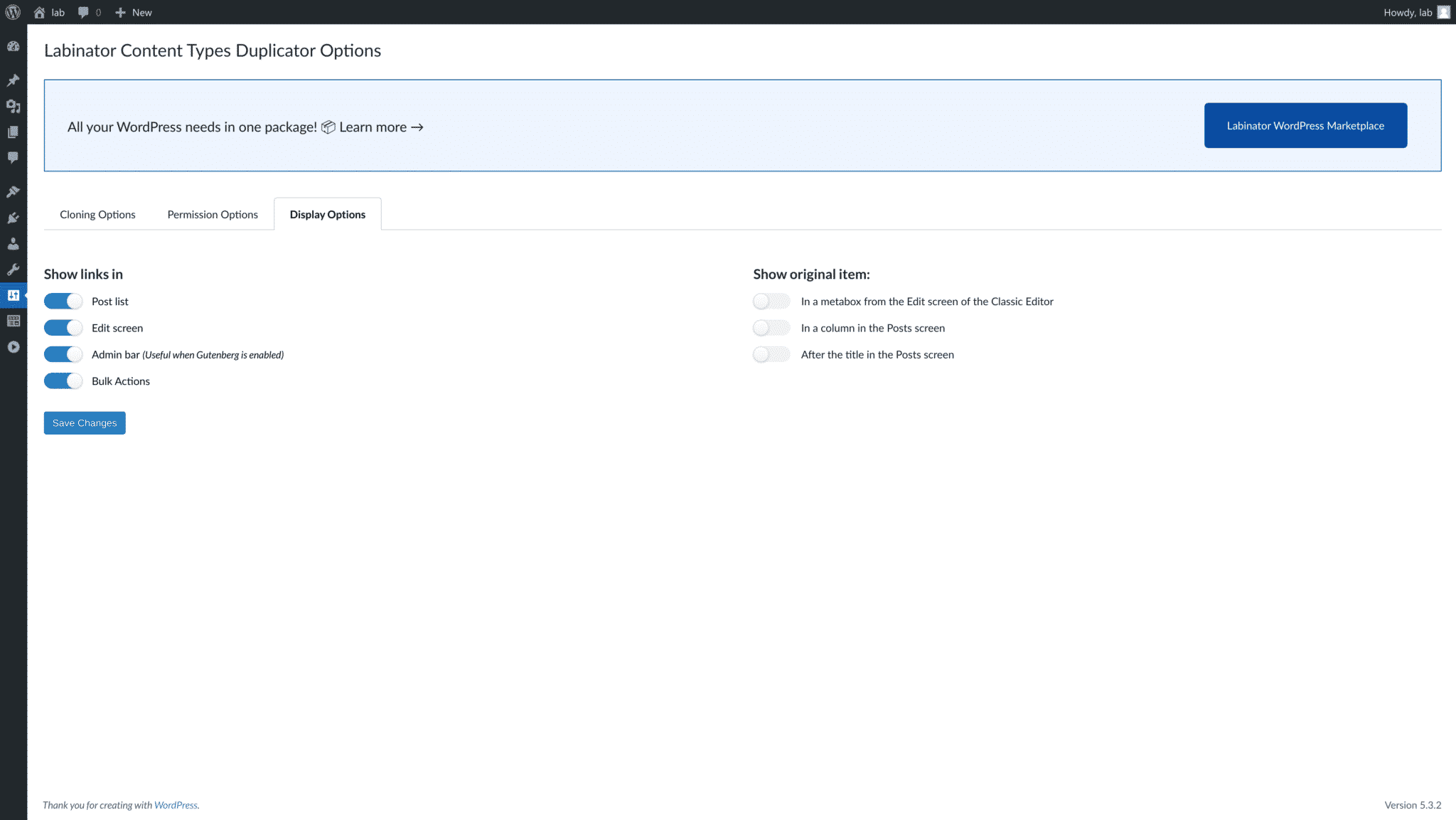This image depicts a webpage application interface framed by a black bar along the left side and top of the page. This black bar houses various icons and buttons, offering multiple functionalities that users can click on. The top right corner features a user account tab for profile management. Directly beneath this area, the application displays a distinct section with bold labels including "Laminator Content Types" and "Duplicator Options."

A prominent blue box is featured at the top of the white section of the page, containing the message "All your WordPress needs in one package. Learn more" alongside a clickable blue button. Below this message are three distinct tabs labeled for "Closing Options," "Permission Options," and "Display Options."

Further down, there are clickable toggle switches allowing users to turn various features on or off. These include a "Show Links" option and, to the right, an option labeled "Show Original Items" with three associated toggle tabs. Overall, the interface appears to be user-friendly, providing easy access to various WordPress settings and customization options.